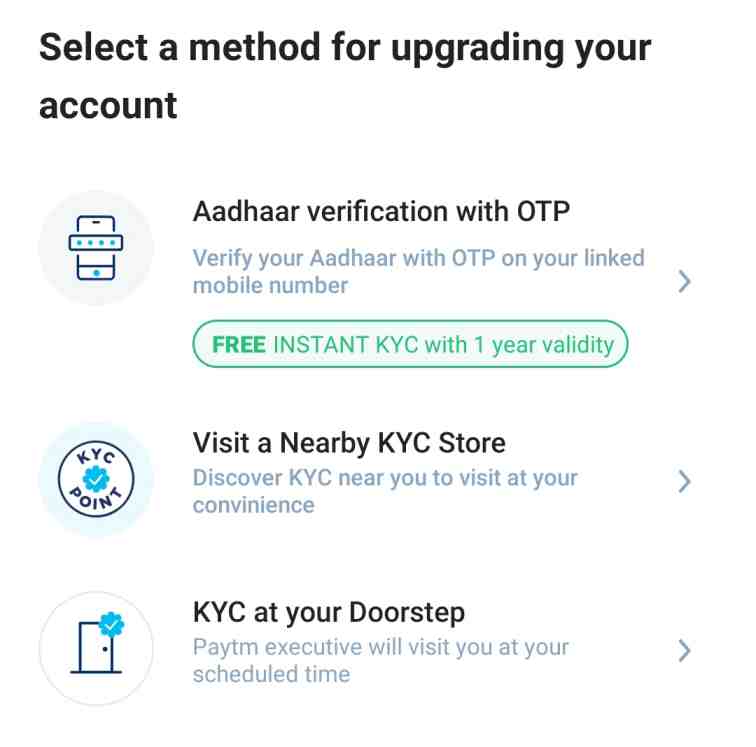The image displays a webpage with options to upgrade an account through various KYC (Know Your Customer) methods. The first option is "Aadhaar Verification with OTP," where users can verify their Aadhaar number—an identification system in India—by using a One-Time Password (OTP) sent to their linked mobile number. Below this option, a green-outlined box highlights, "Free Instant KYC with One Year Validity." 

The second option suggests visiting a nearby KYC store, with the prompt "Discover a KYC store near you to visit at your convenience." 

The third option offers "KYC at Your Desktop," where a Paytm executive will visit the user at a scheduled time to complete the process. 

The overall design has a white background with black text. KYC is a standard procedure for verifying the identity of clients, and the presence of the word "Aadhaar" suggests that this service might be targeting users in India.